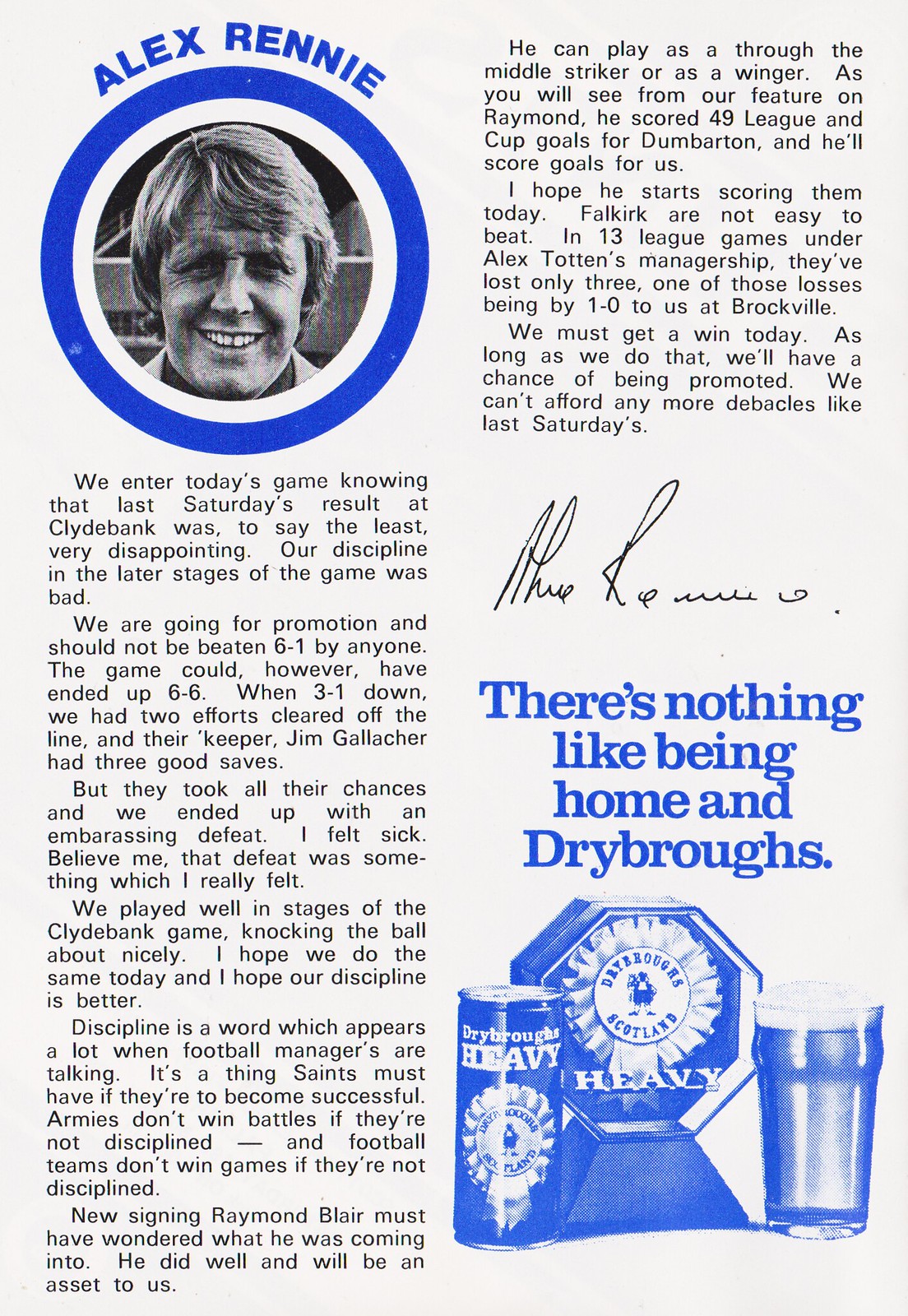This is an image of a page from an old British football magazine featuring a black-and-white photograph of Alex Rennie, a football player, in the top left corner. The photo is circular with a blue outer border and a white inner border, and the name "Alex Rennie" is written in blue capital letters along the curved edge. Rennie, a white man, is seen smiling and slightly squinting, with long hair reaching the back of his neck.

The article text begins with a detailed account of a recent disappointing match result, stating, "We enter today's game knowing that last Saturday's result at Clydebank was, to say the least, very disappointing." It continues to discuss the team's poor discipline and their goal of promotion, emphasizing the critical role discipline plays in success, likening it to armies needing discipline to win battles. The article also highlights new signing Raymond Blair and his expected contributions to the team's success.

Adjacent to the article is Alex Rennie's signature. Below the article, in the bottom right corner, there is an advertisement featuring a stylized drawing of a can and a glass of beer branded "Drybrough's Heavy." The ad, colored in blue, includes the slogan "There’s nothing like being home and dry with Drybrough's," accompanied by images of a trophy-shaped container and a ribbon logo reading "Drybrough's Scotland."